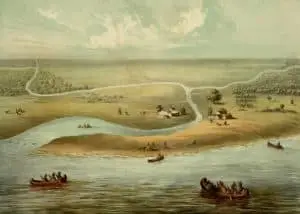This painting, depicting a tranquil 1800s frontier scene, is rectangular in shape and features a subdued palette of neutral colors. The sky is a blend of bluish-white, creating a serene backdrop for the image. The composition centers around a river which winds from the foreground towards the middle top, branching off into tributaries that stretch towards the far left and right corners. The water is a muted blue, bordered by a small green and beige peninsula jutting into the scene. Various canoes, each carrying two to three people, dot the river and its tributaries, providing a sense of activity.

The land, primarily bare with patches of green and brown grass, is sparsely populated with small structures and homes, possibly huts, that stand faintly against the landscape. Scattered small trees are visible on either side of the land mass, adding a touch of vegetation to the scene. To the left background, there is a suggestion of a forest without clearly defined trees. Overall, the painting captures a serene moment of everyday life along the river, with its delicate details and soft color scheme contributing to a nostalgic and peaceful atmosphere.